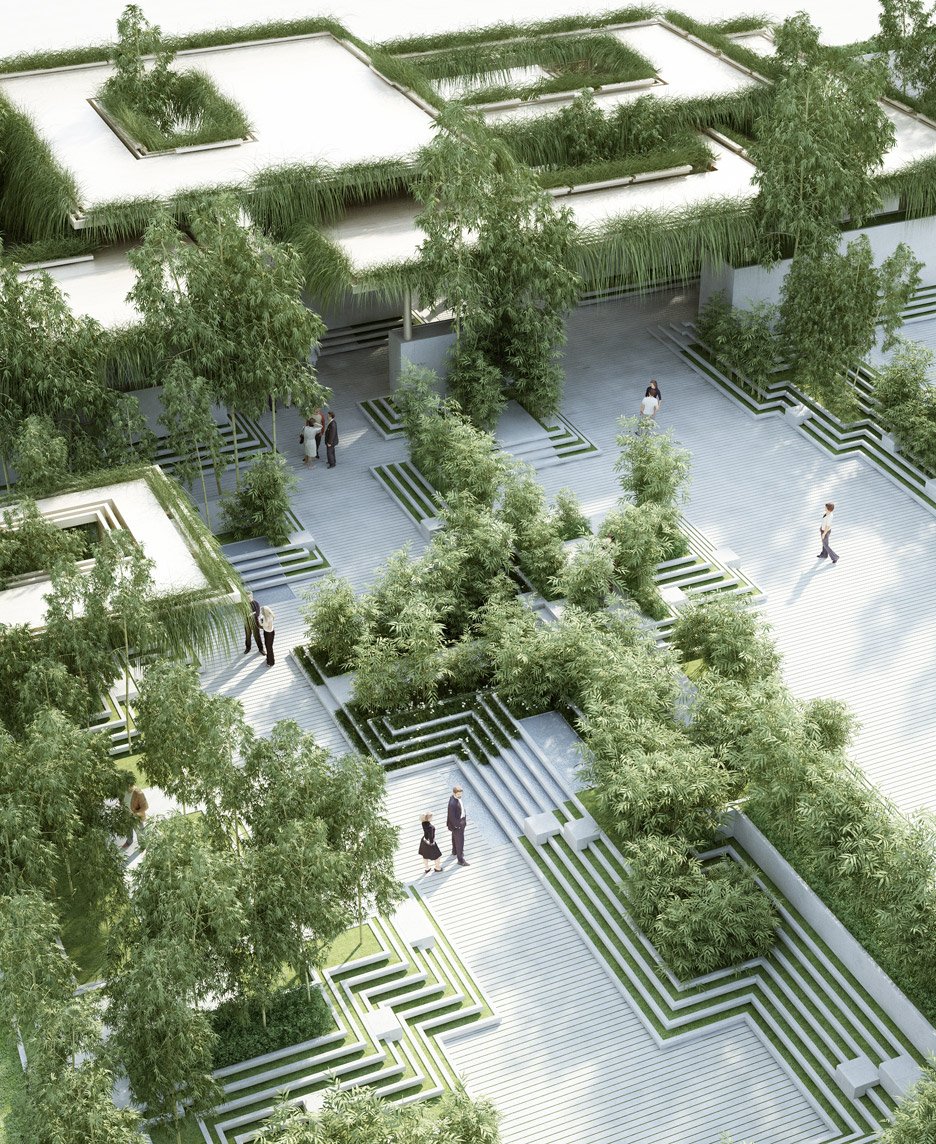This image is an aerial perspective of a lush, multi-layered park, appearing almost like a digital creation. The park's unique design features various levels and terraces, each adorned with vibrant shades of green from trees, grasses, and shrubs. The pathways, which appear to be made of wood, zigzag through the park, creating a harmonious blend of angular segments of lawn and natural elements. Scattered throughout these paths and terraces are ten people, including a man in a suit and a woman in a dress, providing a sense of scale and activity within the space. The park's architectural elements also include buildings with rooftop gardens, featuring pathways lined with ornamental grasses. The predominant colors in the image are diverse greens, browns, whites, blacks, and sky blues, enhancing the vivid and serene atmosphere of this meticulously designed landscape.